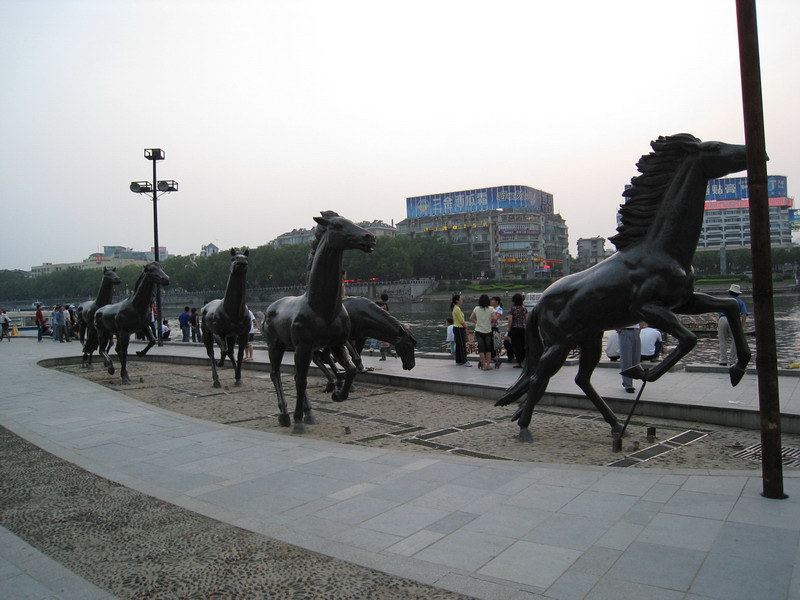The photograph features a striking sculpture of six dark metal horses arranged in a dynamic composition that suggests movement, with their poses ranging from rearing up on hind legs to galloping. The horses are positioned on a slightly sunken platform, surrounded by light gray brickwork. Positioned diagonally, the statues appear larger on the right and taper towards the left. Behind the sculpture, people gather along the edge of what appears to be a river or canal, some crouching and others standing in small groups. The background showcases a scenic view with trees and two prominent buildings across the water, each adorned with signs featuring white Asian lettering on a blue background. A large pole stands near the right side of the composition, adding to the depth of the scene.